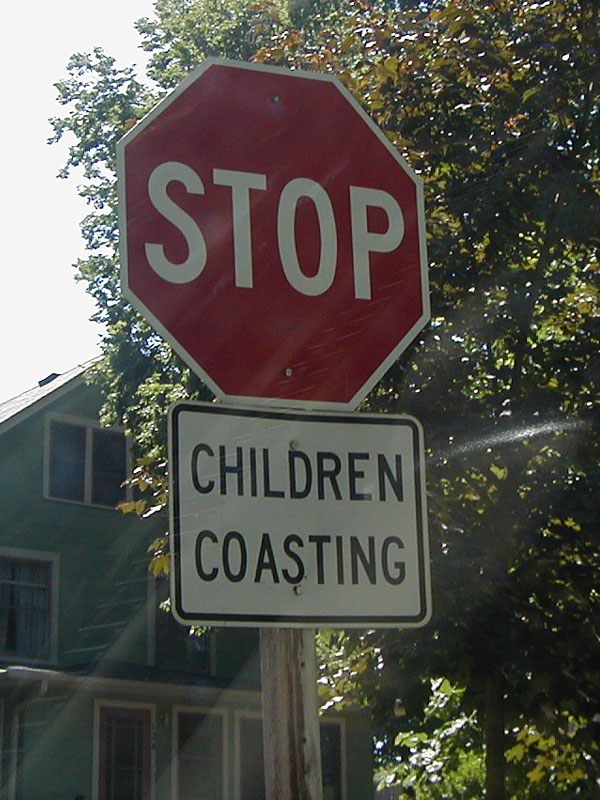In the foreground of this image stands an octagonal red stop sign with the word "STOP" prominently displayed in white lettering and outlined in white. Directly beneath it is a rectangular white sign bordered in black, bearing the capitalized message "CHILDREN COASTING." Both signs are mounted on a gray pole, indicating a cautionary warning for drivers in the area.

The scene is set in a residential neighborhood, characterized by a house in the background. The house features a greenish exterior and is notably detailed with multiple windows: four on the first floor, two on the second floor, and three small rectangular windows at the very top. These various details provide a glimpse into the architectural style prevalent in the neighborhood.

The lighting suggests a bright day, with the sun creating a glare on the stop sign and a high exposure area in the top left corner of the image. However, the overall light quality seems diffused, possibly hinting at a recent storm or overcast conditions. Adding to the residential feel, tree leaves and branches are visible to the right of the sign, contributing to the natural ambiance of the scene.